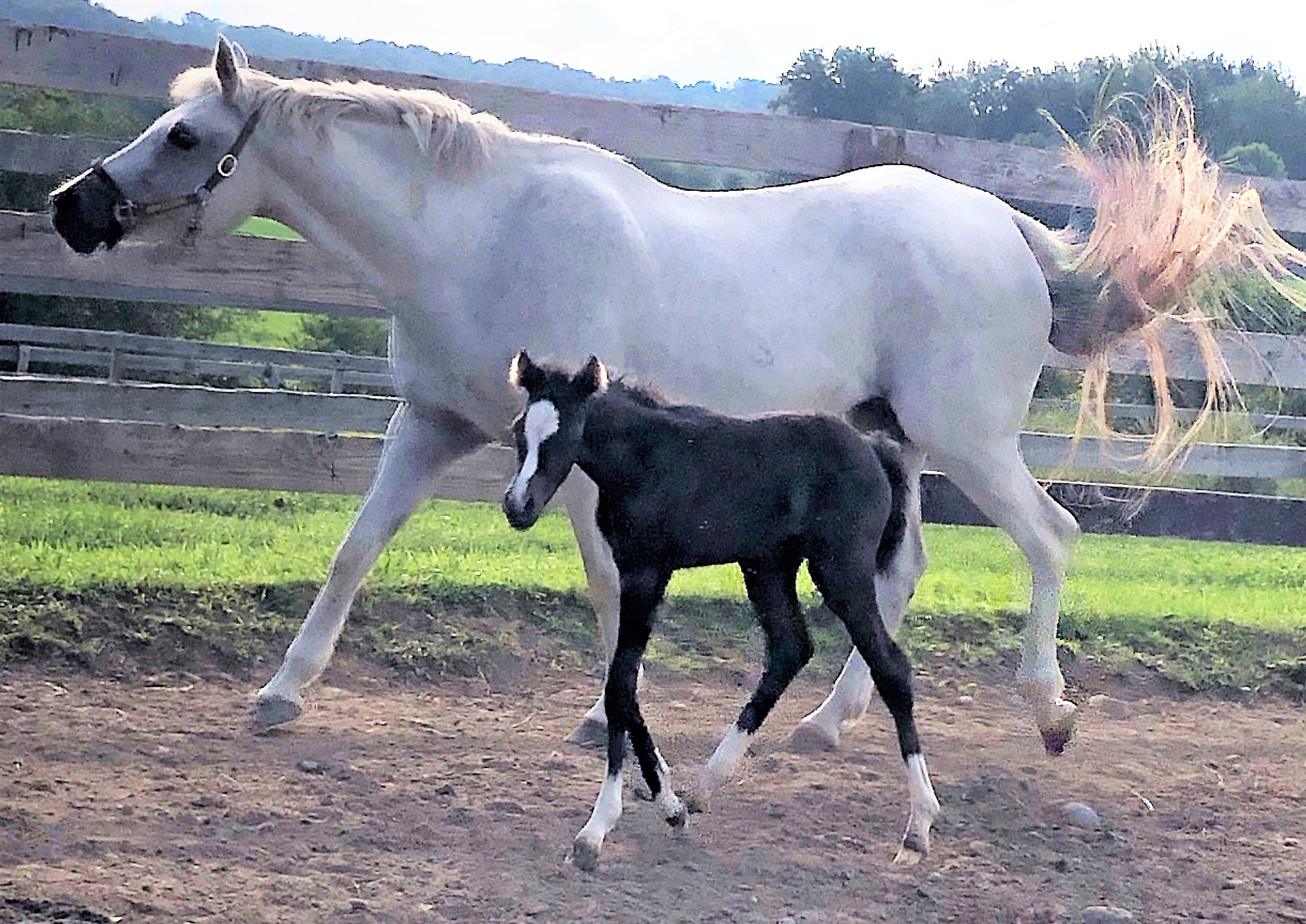In this vividly detailed photograph, a majestic adult white horse and a young black foal are captured in graceful motion, galloping together under the bright daylight. The adult horse, much larger in size, possesses a flowing, bushy white mane and a tail that shimmers with a creamy hue, tipping into a slightly peachy color. Adorned with a black muzzle around its nose and mouth, the horse's mane and the raised tail suggest dynamic movement across the dirt path they traverse. Beside the adult horse trots the little foal, predominantly black with distinctive white markings: its ankles appear as white "socks," and it brandishes a spoon-shaped white blotch on its forehead. The foal is estimated to be one or two years old and mirrors its mother’s stride with youthful energy. Behind the horses stands a sturdy wooden fence, painted either white or light brown, enclosing a verdant field of meticulously mowed, bright green grass. The backdrop further includes a row of deciduous trees and distant mountains, adding depth and natural beauty to the scene. The sky overhead is bright and seemingly white, bathing the whole setting in a brilliant daylight glow.